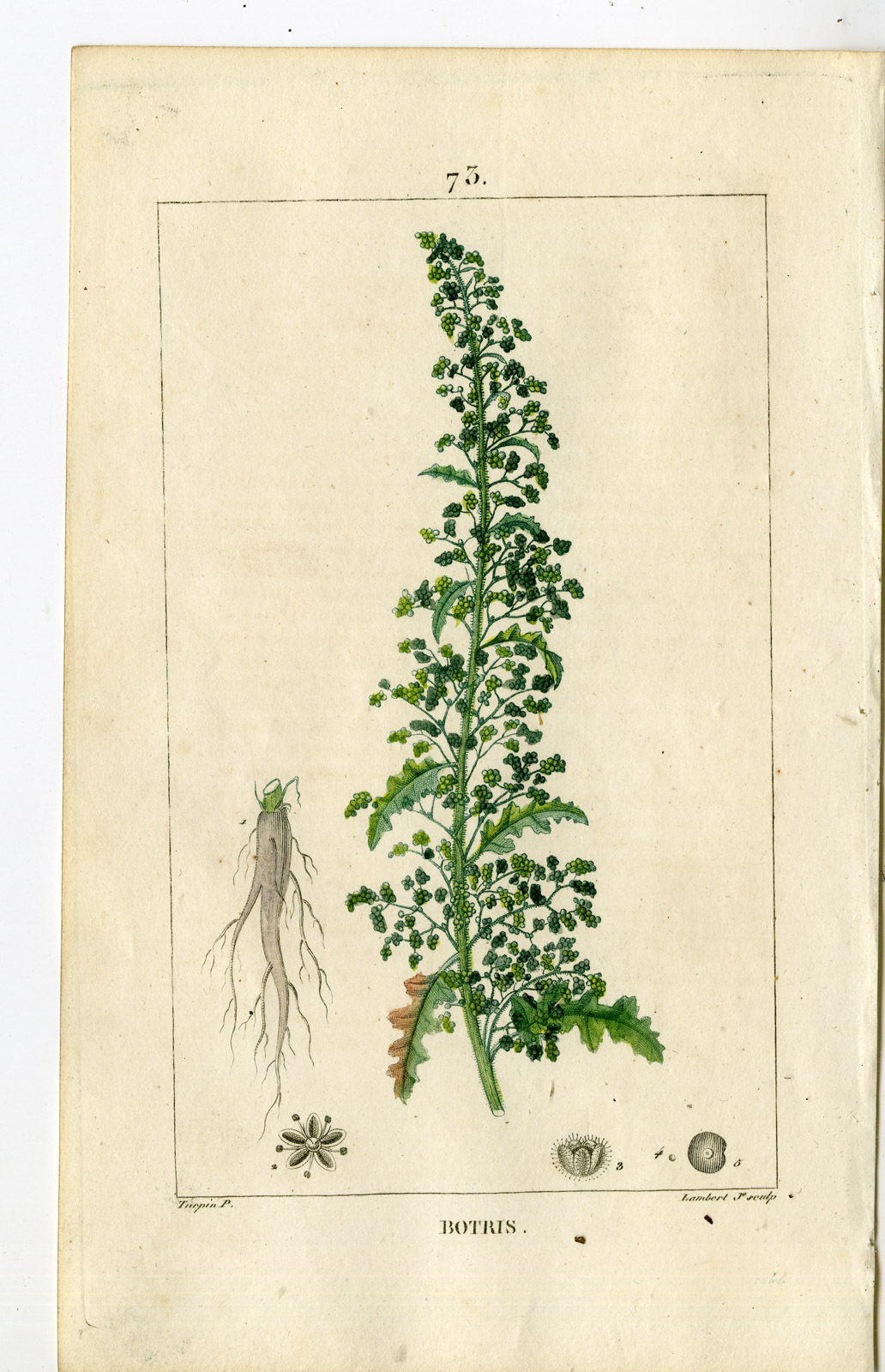The image in question is a detailed, vertical rectangular print, likely taken from an old book, indicated by its aged off-white paper with yellow stains. It features a thin black outline and a light gray border along the top and left edge, with a number 75 at the top and the word "Botris" at the bottom. The central illustration depicts a tall, green plant with a slightly wavy stem. Numerous thin green branches extend from it, adorned with small, spiky-edged leaves and numerous tiny green buds resembling berries. To the left of the plant, the root system is illustrated in black and white, showing a primary long gray root tapering to a point with thinner stringy roots branching out. The bottom of the image includes three small geometric shapes in gray, adding to the diagrammatic nature of the piece.